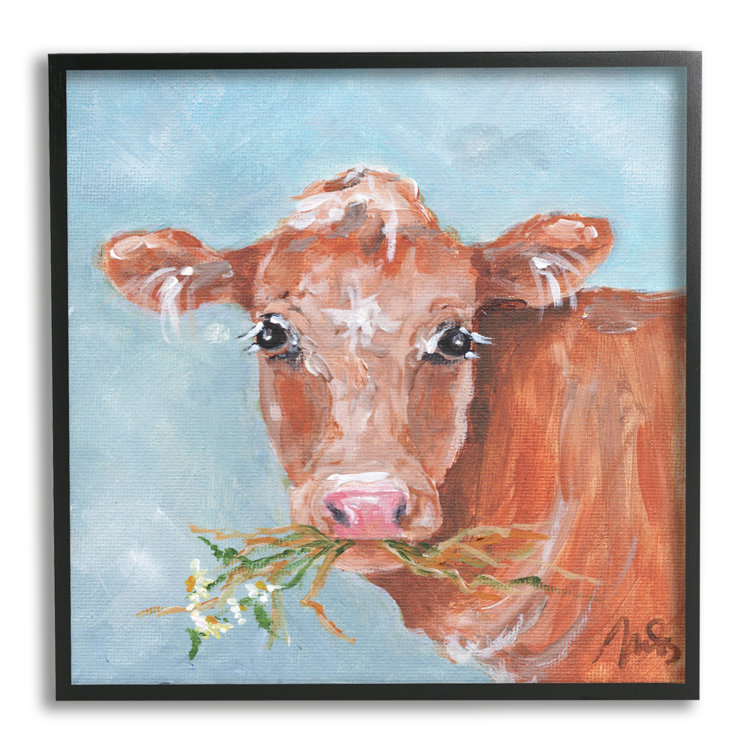The image depicts a square, oil or acrylic painting of a young, brown Jersey cow, distinctively framed by a simple, thin black border. Dominating the center of the composition, the cow's head is turned to face the viewer directly, while its neck and front flanks extend off to the right. The cow, with its small face, big dark eyes, and long eyelashes, displays pointed ears adorned with white tufts of hair. A mouthful of daisies, complete with stems and leaves, is held horizontally, sticking out both sides of its mouth. The background reveals a mottled blue sky, providing a simple yet effective contrast to the cow. An artist's signature is positioned in the lower right corner of the painting.